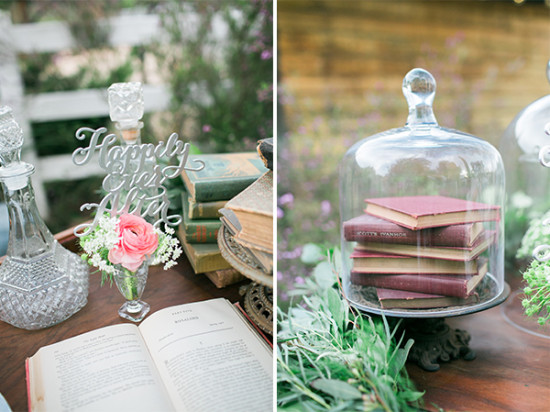This image is divided into two equal-sized rectangles, each showcasing a different scene. 

In the left picture, set outdoors on a wooden table, there is a small vase with a pink rose and possibly a carnation, surrounded by flowers. Above the vase, the words "happily ever after" are displayed in gray, possibly attached to a stick or resting on a surface behind the flowers. Beside the vase, there is a crystal chalice or decanter with a cork. In front of the vase, an open book lies on the table, with a stack of books, including green hardbacks, to its right. The background includes a white fence and some bushes, adding to the serene outdoor ambiance.

The right picture features a cake stand with a domed glass cover, inside which six books with reddish-maroon covers are neatly stacked. The stand appears to have a wooden base. Surrounding the cake stand are various flowers and leaves, with a wall and grassy plants visible in the background, contributing to the overall aesthetic of a wedding celebration setup.